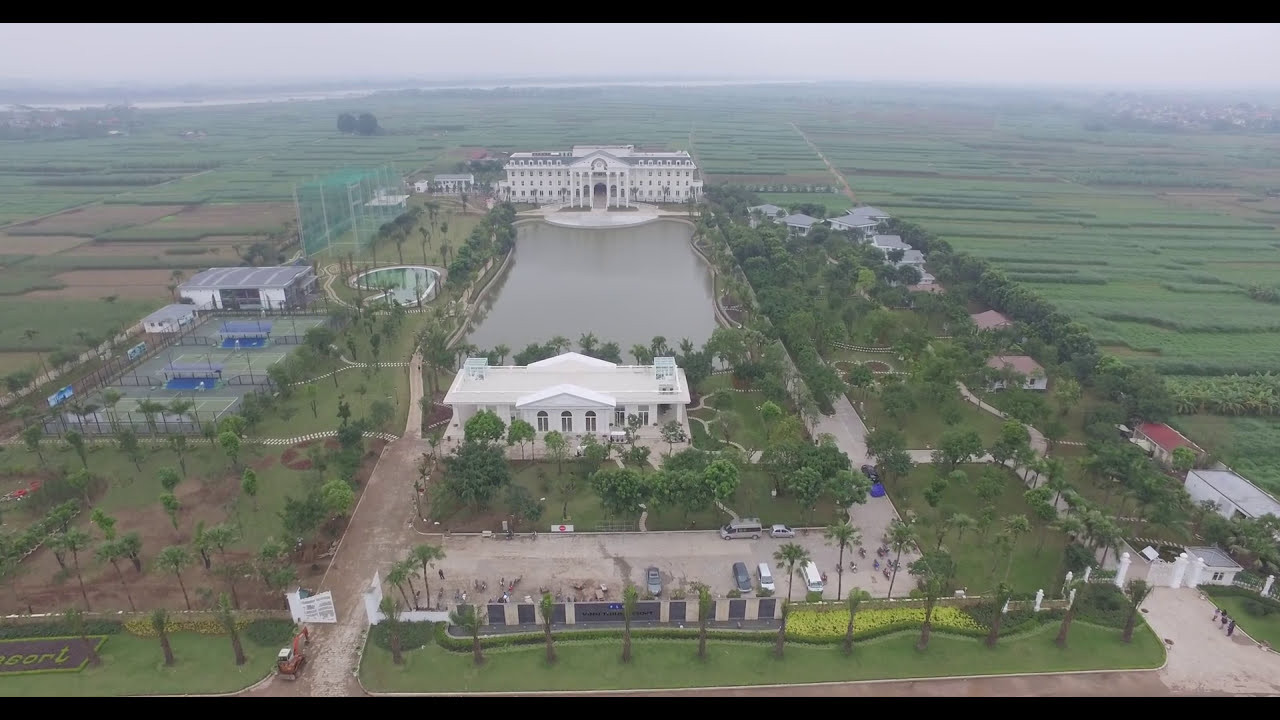The photo captures an expansive, lush green estate viewed from an aerial perspective, framed by thin black bars at the top and bottom. Dominating the image is a grand white mansion with a classical architectural style, featuring six tall white columns at its grand entrance. A circular driveway leads up to the mansion, emphasizing its stately presence. Directly in front of the mansion lies a large, square reflecting pool with rounded edges, adding to the estate's opulent feel. Beyond the pool stands another sizable white building, its back adorned with arched windows in the center flanked by regular large windows.

To the left of the image, three tennis courts and a swimming pool can be seen amidst the manicured grounds. A gym-like building and what appears to be several football fields with blue seating are also visible. Scattered throughout the estate are numerous trees, short grass walkways, and various smaller buildings.

The right side of the property features a gatehouse and a car park with a few silver and white cars. A digger is working on a pathway near an open gate. Surrounding the gate and fencing are tropical trees adding a touch of exotic appeal. Beyond the immediate estate, the landscape transitions into farmlands and plantations, with a river and a distant town visible at the top right of the image.